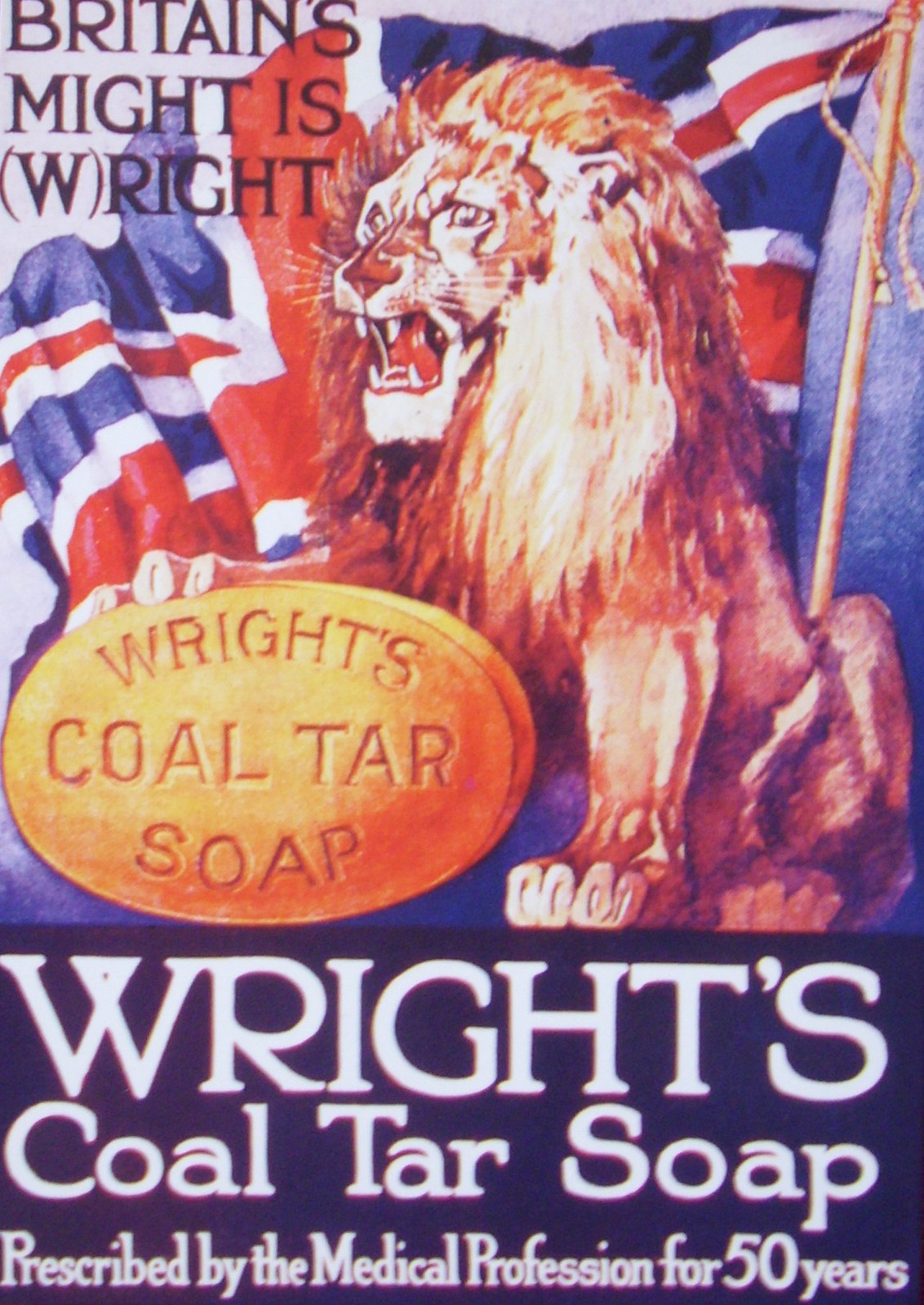The image is an old-fashioned advertisement for Wright's Coal Tar Soap. The upper half features a detailed illustration set against a light blue background. A majestic lion with a gold mane and white face sits on its haunches, roaring, and is positioned slightly to the right. Behind the lion, a flagpole extends from the right towards the left, displaying a furled British flag in red, white, and blue. The text "Britain's might is right" with a stylized "W" in parentheses, is prominently displayed in the upper left corner in dark print.

Directly below the lion's open mouth, its right paw rests on an oval-shaped bar of soap. The soap is depicted in a golden yellow color, with the text "Wright's Coal Tar Soap" in gold inset. Further down in the image, a deep blue stripe spans the width, featuring the same text, "Wright's Coal Tar Soap," in white print. At the very bottom, it reads, "Prescribed by the medical profession for 50 years," underscoring the product's long-standing endorsement.

The entire composition is arranged within a vertical rectangle, with the lion centered towards the right and the soap positioned slightly left of center, maintaining a balanced yet dynamic layout typical of classic, vintage advertisements.